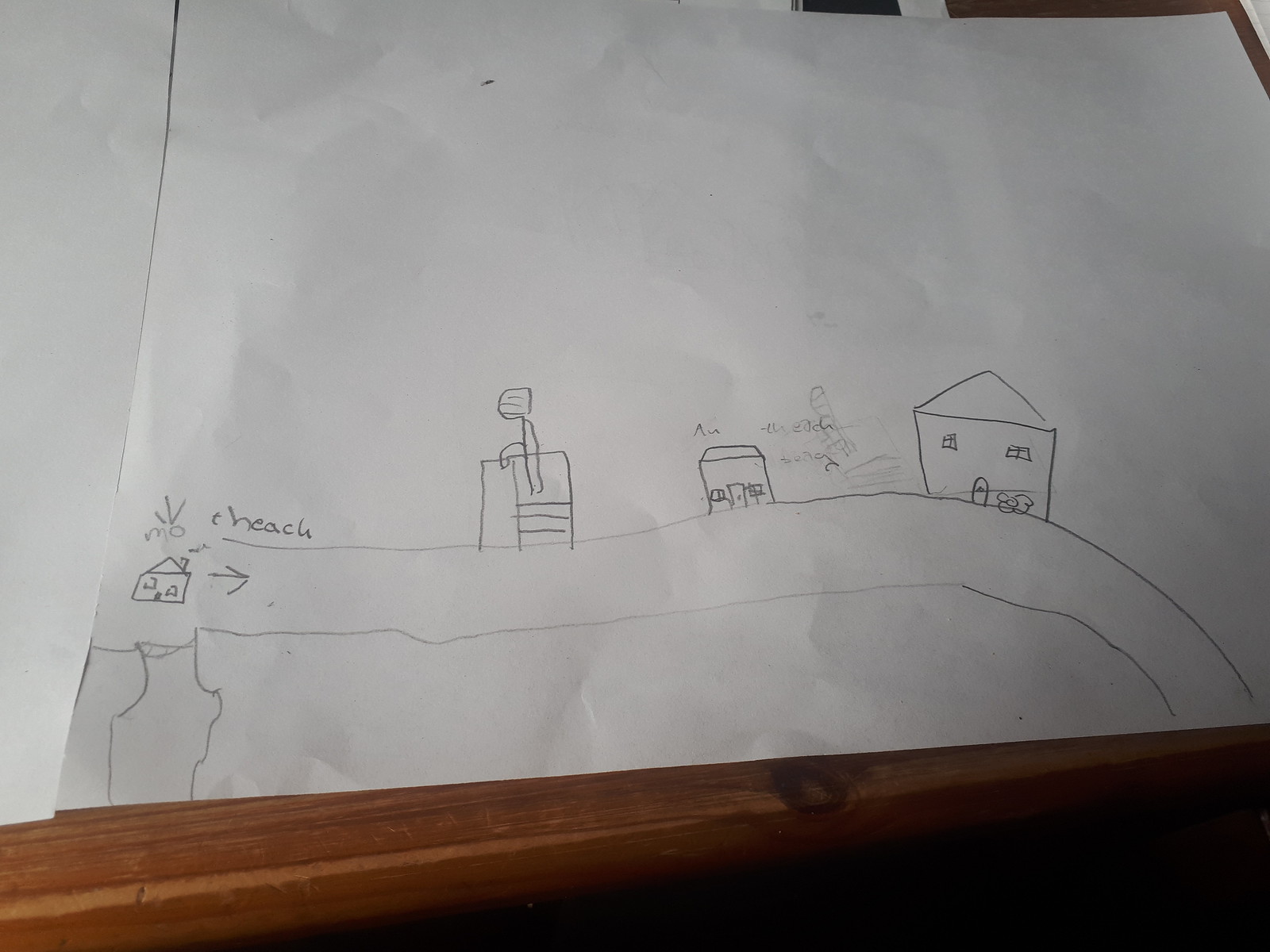The image depicts a children's hand-drawn picture, rendered in pencil on a large piece of paper, which is placed atop a wooden table or desk. The central element is a narrow road, sketched using two parallel strokes of the pencil. On the road, there's an almost erased word with an arrow, which might have said "beach" at some point. 

Towards the upper part of the picture, there is a small house with an arrow pointing down the road. Along this road, a simplistic figure is depicted climbing stairs, seemingly going down a slide. The figure consists of two lines for the body, a circle for the head adorned with several lines, and a singular, hook-like arm.

Additionally, a second house with a flat roof appears in the drawing. This house is surrounded by numerous eraser marks, indicating changes or corrections. Further along the bend of the road, a larger house is prominently featured. At the road's start, wavy lines extend vertically from the house, leading down to the paper's edge.